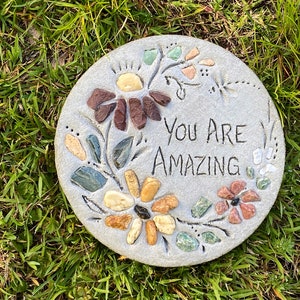The image depicts a handmade, round stepping stone or clay mold, set against a background of green grass and brown dirt with no other objects present. The stone lies flat on the ground and is adorned with a heartwarming message in all capital letters, "YOU ARE AMAZING." This text is surrounded by a colorful floral design that includes a variety of flowers with purple, orange, yellow, and pink petals, as well as green leaves and a vine encircling the stone. Additionally, a small firefly is incorporated into the design. The stones and flowers look hand-painted and intricately detailed, suggesting that it might be a DIY project using rocks to form the floral elements. The perspective of the image is a bird's-eye view, emphasizing the detailed craftsmanship and vibrant colors of the object.